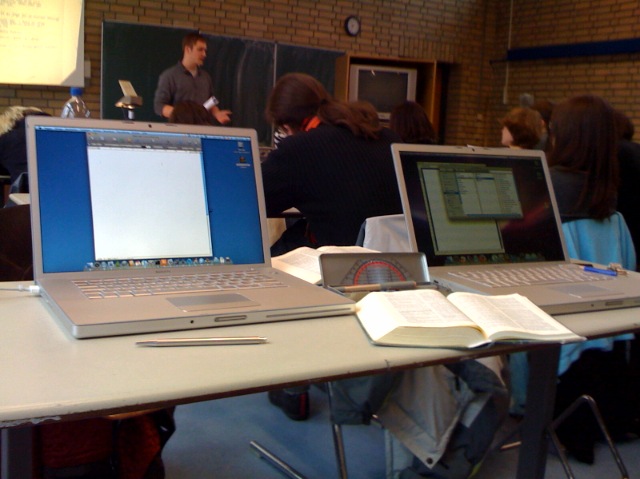The image captures an older classroom setting, likely from 2003 or earlier. It features a man at the front, possibly a professor, wearing a gray button-up shirt, gesturing emphatically with both hands as he lectures. The classroom has a noticeable brick wall adorned with a classic black-and-white wall clock and a green blackboard. There is also an old CRT TV mounted on the right side of the room. 

In the foreground, a long desk accommodates several students sitting side by side. On this desk, there are two early Apple laptops—possibly iBooks or early MacBooks—alongside an open book and a thin silver pen or stylus. One laptop displays a blue screen with an open web page or a blank page, while the other, slightly blurred, shows a dark screen with some information. In front of the professor, more students can be seen; one appears focused with their head down, taking notes, while another looks up attentively at the instructor. The scene suggests an engaging educational environment from over a decade ago, highlighting both the technology and classroom dynamics of that time.